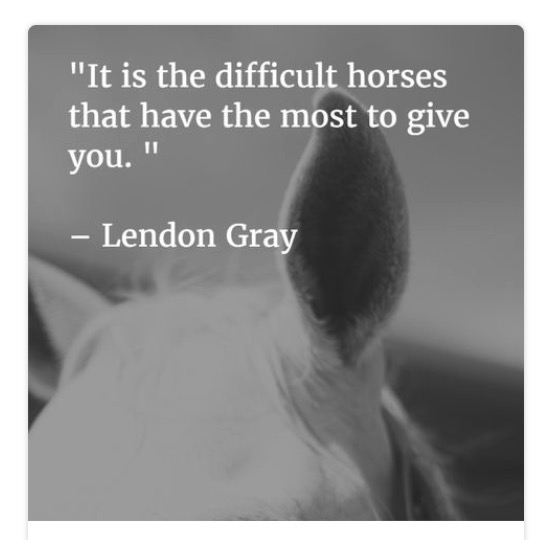This is a black-and-white square image featuring a poignant quote prominently left-aligned at the top. The text reads, “It is the difficult horses that have the most to give you," followed by a dash and the name "Lendon Gray." The background behind the text appears blurred and gray, resembling a wall or possibly a dark field. The lower half of the image reveals the partial head of a horse with a white mane. The ears, centrally positioned and pointed towards the viewer, have a gray exterior and black interior. The corners of the image are rounded, enhancing its modern aesthetic. The composition clearly emphasizes the wise words of Lendon Gray paired seamlessly with the softly focused imagery of the horse, symbolizing depth and insight.